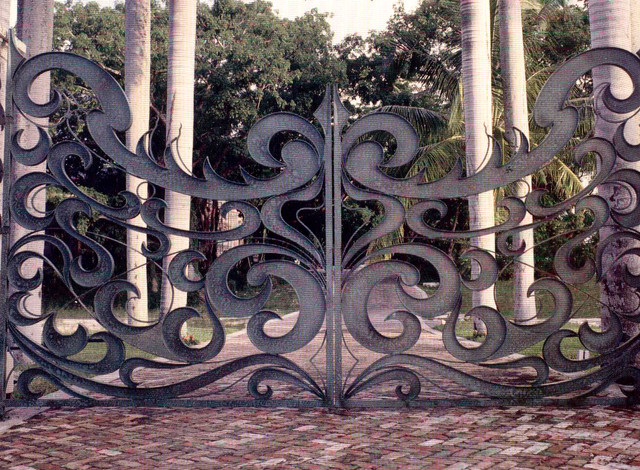This photograph prominently features an elaborate wrought iron gate that dominates the image. The gate consists of two swinging halves that meet at the center of a brick pathway. Intricately designed with swirling and crescent moon shapes, most of its space is left open, allowing views through to the background. The gate appears dark purple, though it also has been described as silverish-gray or black, indicating possible varying lighting or color perception. 

The path beneath the gate is composed of bricks in various shades, from rose to purple to violet. Flanking the gate on either side are tall, narrow tree trunks with purplish-white or white cream-colored bark, stretching out of the frame. In the background, a canopy of green foliage is tinged with a purple hue, suggesting a filter effect. The far background fades into darkness, hinting at a dense forested area. Grass lines both sides of the brick pathway, adding to the natural setting.